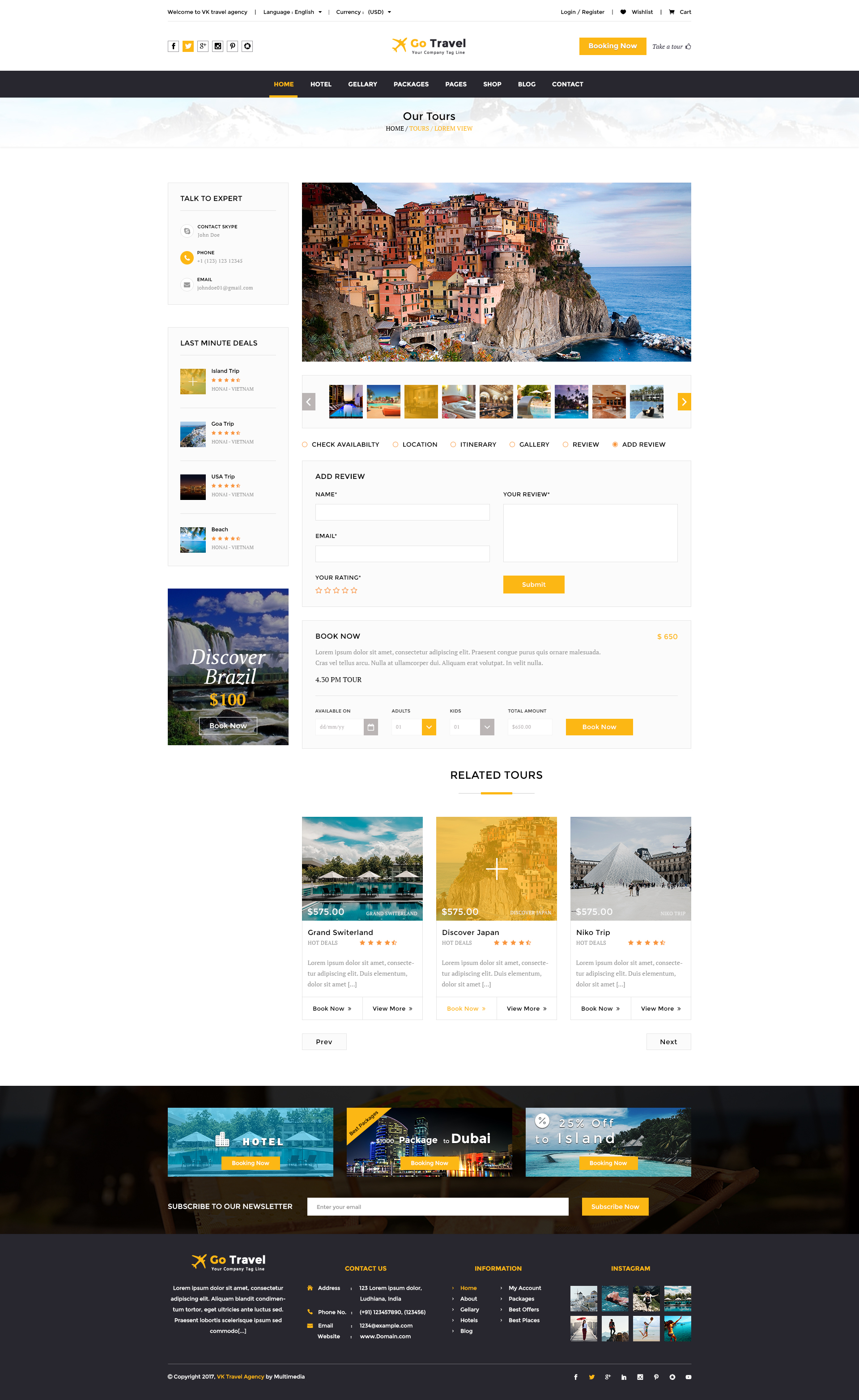This screenshot captures the entire webpage of the "GoTravel" website. The top section features five social media icons, with one highlighted in gold and the others in monochrome. Centered prominently is the "GoTravel" logo, which includes a gold airplane icon. Below the logo, "GoTravel" is written again. To the right of the logo is a gold rectangular button with white text inside it, followed by additional text.

Beneath this header, there is a black navigation bar with several underscored, gold-highlighted sections, possibly starting with "Home," and continuing with seven other selections. Directly below this is a section titled "Art Tours," accompanied by an image likely depicting a European, possibly Italian, destination, and smaller related pictures on the side. 

Further down, there is an area for users to fill out information. The left-hand sidebar contains small media images with ratings. At the bottom of the page, there's a section labeled "Related Tours" featuring more media images. The footer includes another black banner with additional media images, a search bar, and further information about "GoTravel."